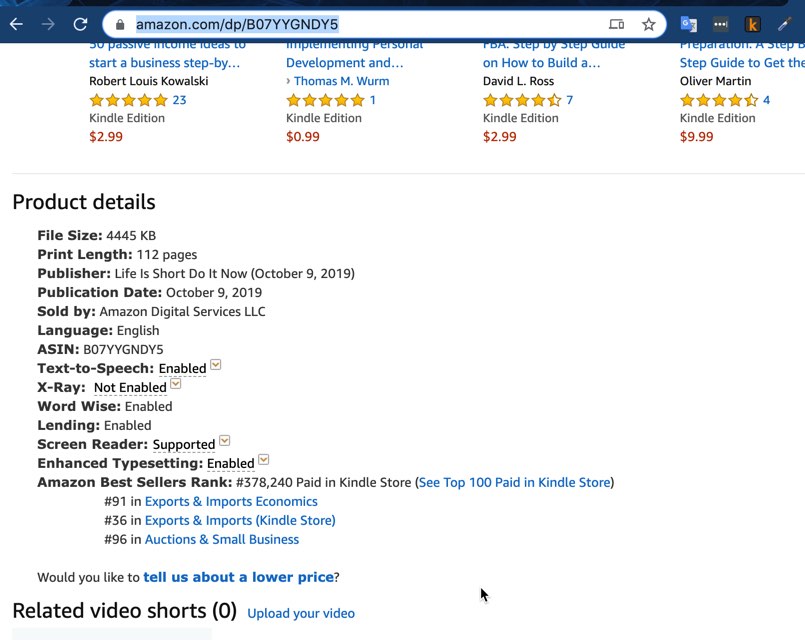In the image, a user is browsing a specific page on Amazon and has scrolled down to the 'Product Details' section. The page highlights the details of a digital book, which spans 112 pages. The title of the book is not visible, but it is evident that the publisher is "Life is Too Short, Do It Now," and the publication date is October 9, 2019. The book supports screen readers and features enhanced typesetting. Additionally, related products shown above the details suggest that the book falls within the self-help or finance genre, possibly a non-fiction guide focused on step-by-step methods for generating passive income. The Amazon bestseller rankings hint at its association with economics and small business categories.